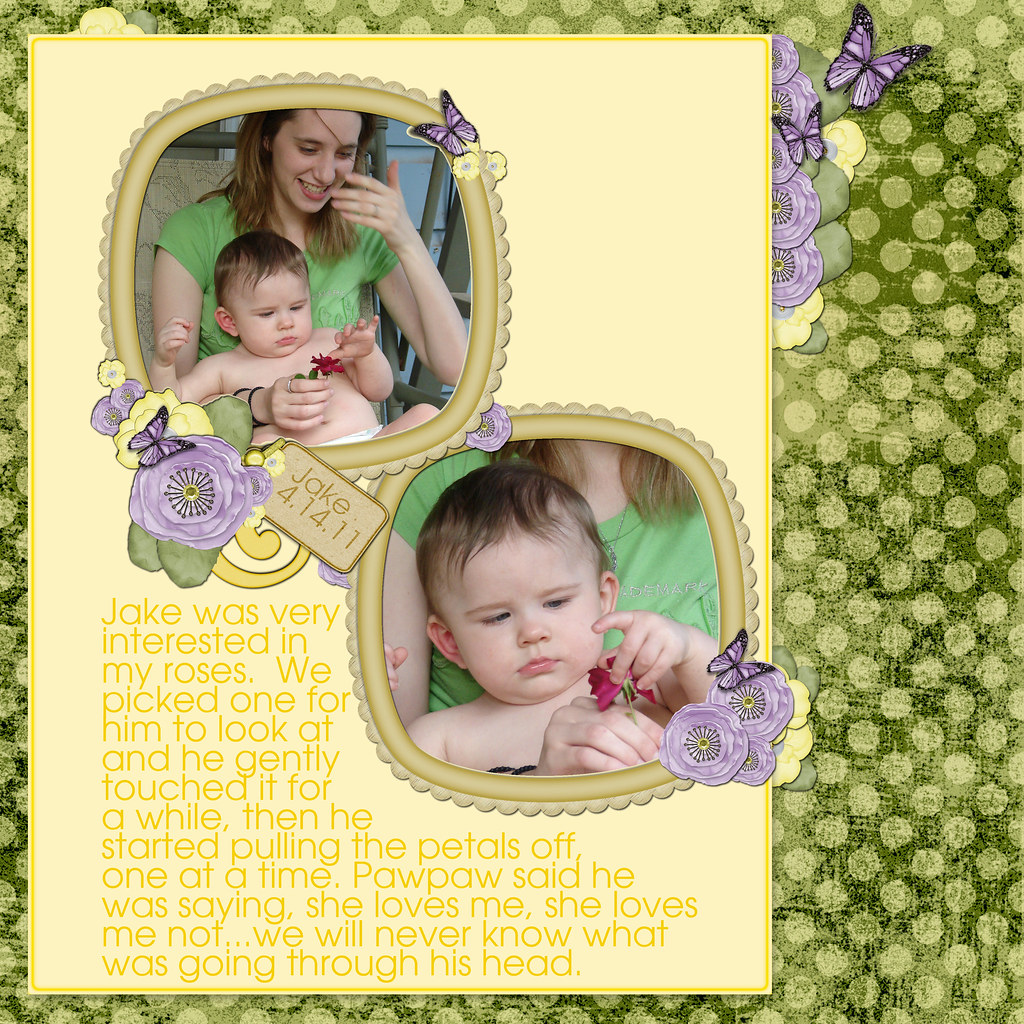In a light yellow scrapbook-style graphic with a grungy polka dot green background adorned with little purple flowers and butterflies, two photos capture a tender moment between a Caucasian mother and her baby, Jake, dated April 14, 2011. The woman, wearing a green shirt, looks amused as she holds her diaper-clad baby, who interacts with a magenta rose. Jake initially touches the rose gently before methodically pulling off its petals, perhaps mimicking the "she loves me, she loves me not" game. This heartwarming scene, set against a creatively decorated backdrop with yellow fonts and an overlay of small flowers and butterflies, encapsulates a precious memory and adds a narrative charm to this scrapbook page.